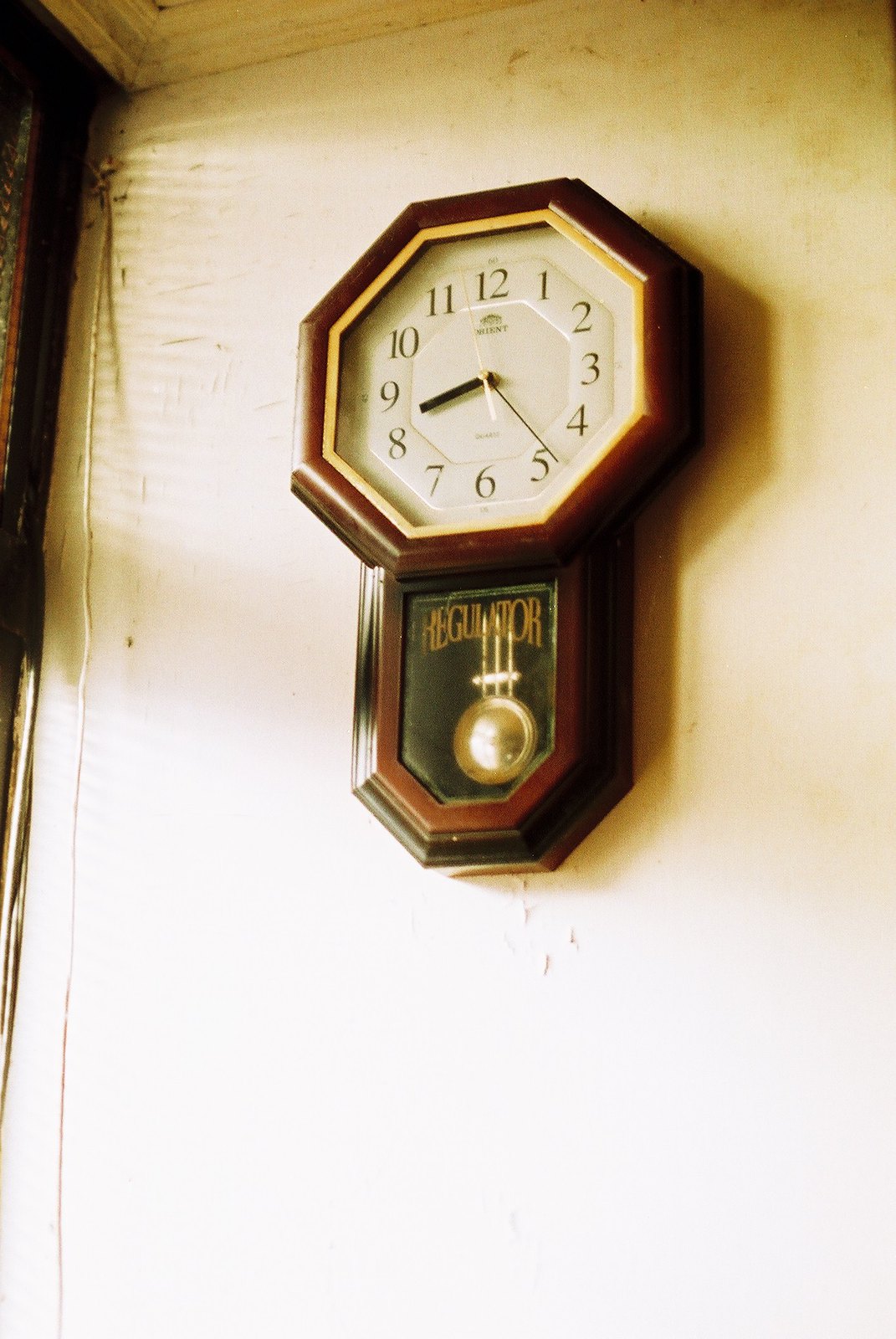The image depicts a distinctive wall-hanging clock with an octagonal shape, elegantly framed in dark brown wood. Below the clock face, a shield-shaped wooden extension features straight lines that taper into a pointed end, enhancing its unique aesthetic. Encased within this ornate wooden frame is a gold-toned pendulum, adding a touch of sophistication. Additionally, three decorative hangers, aligned horizontally near the pendulum, complement the overall design.

The clock face itself is outlined in a gold tone, contrasting beautifully with the white background. It features black Arabic numerals, black minute and hour hands, and a gold-toned second hand for precise timekeeping. This exquisite timepiece is mounted on a pristine white wall, emphasizing its classic and refined look.